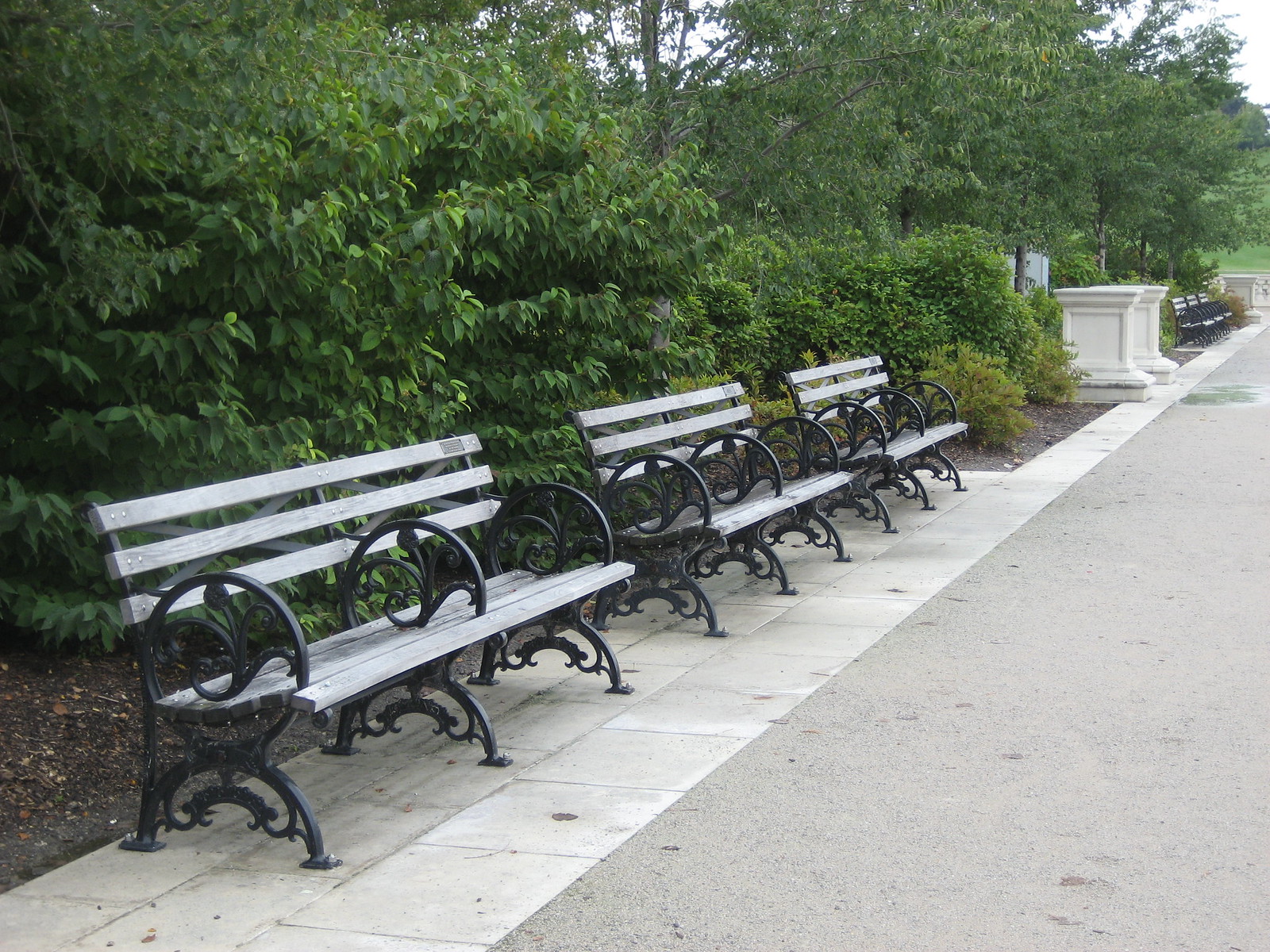This image captures a serene scene in what appears to be a public park or green space, devoid of any visible buildings. It’s a clear, sunny day, with a vivid blue sky free of clouds. Directly in the foreground, three elegantly-designed benches are lined up in a row, positioned along the edge of a stone pathway which extends from the bottom right to the middle of the photo. The benches are crafted from light grey wood slats, providing a rustic charm, and are supported by intricately designed dark metallic frames. The base of each bench features large, circular metal pieces adorned with artistic plant motifs, which elegantly curve upwards and connect to semicircles at the ground level. These benches rest atop large, square marble tiles, bordered by small stone pillars that add to the classic aesthetic of the space.

Behind the benches, a lush row of bright green shrubbery occupies the background, creating a natural barrier that adds depth and vibrancy to the scene. In addition to the large bushes, the background includes tall green trees and ornate stone planter pots nestled against the edge of the pathway. Beyond these planter pots lies another row of identical benches, emphasizing the orderly and symmetrical layout of this peaceful park setting.